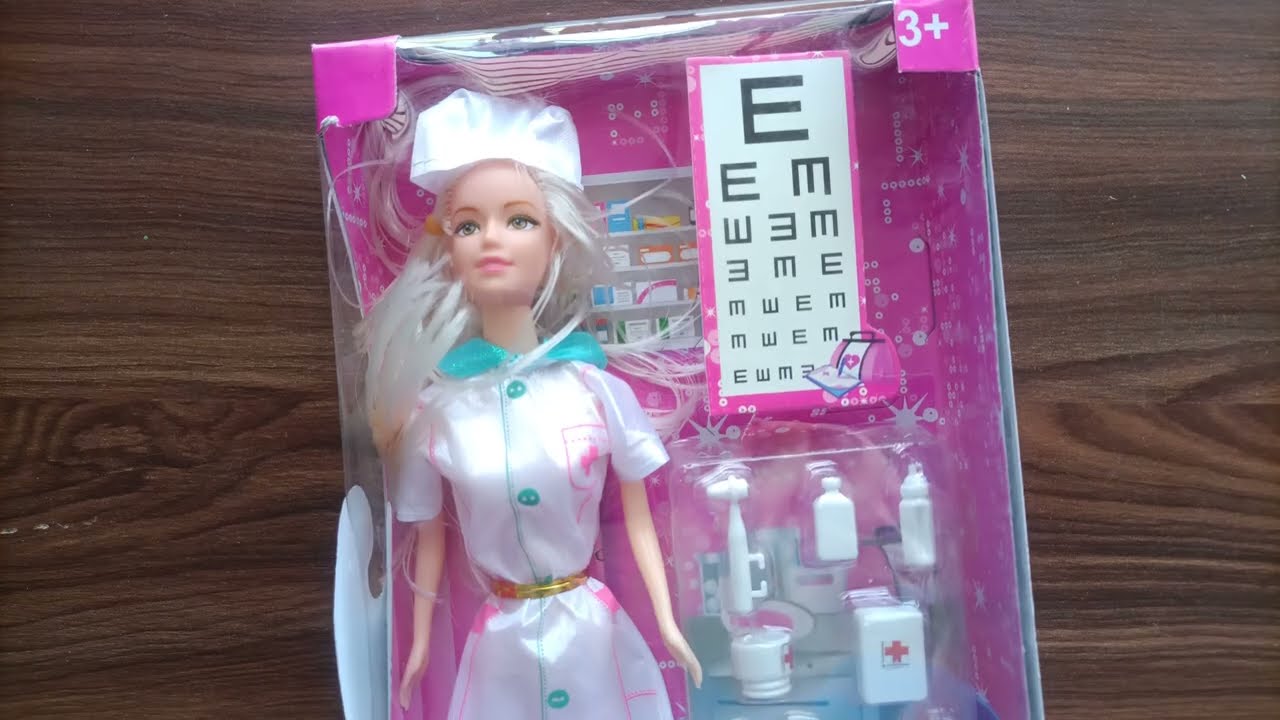In this photograph taken indoors, likely on a child's wooden desk, there is a boxed Barbie set prominently laid out. The wooden table surface, brown in color, completely fills the background of the image. At the center of the image, at a slightly diagonal angle, lies the Barbie, fully encased in its slightly damaged transparent plastic packaging. The Barbie is dressed as a doctor, specifically an ophthalmologist indicated by the distinctive white uniform with a teal collar. Surrounding the Barbie are various small plastic medical instruments, including a cup, bottles, and a box marked with a plus sign. A notable feature inside the packaging is a small board featuring various oriented alphabet 'E's, used to mimic the ophthalmologist's eye chart. The backdrop behind the Barbie inside the packaging is colored pink, adding contrast to the overall presentation. Various shades of brown, pink, black, white, light blue, gray, and red add to the overall color palette of the scene.